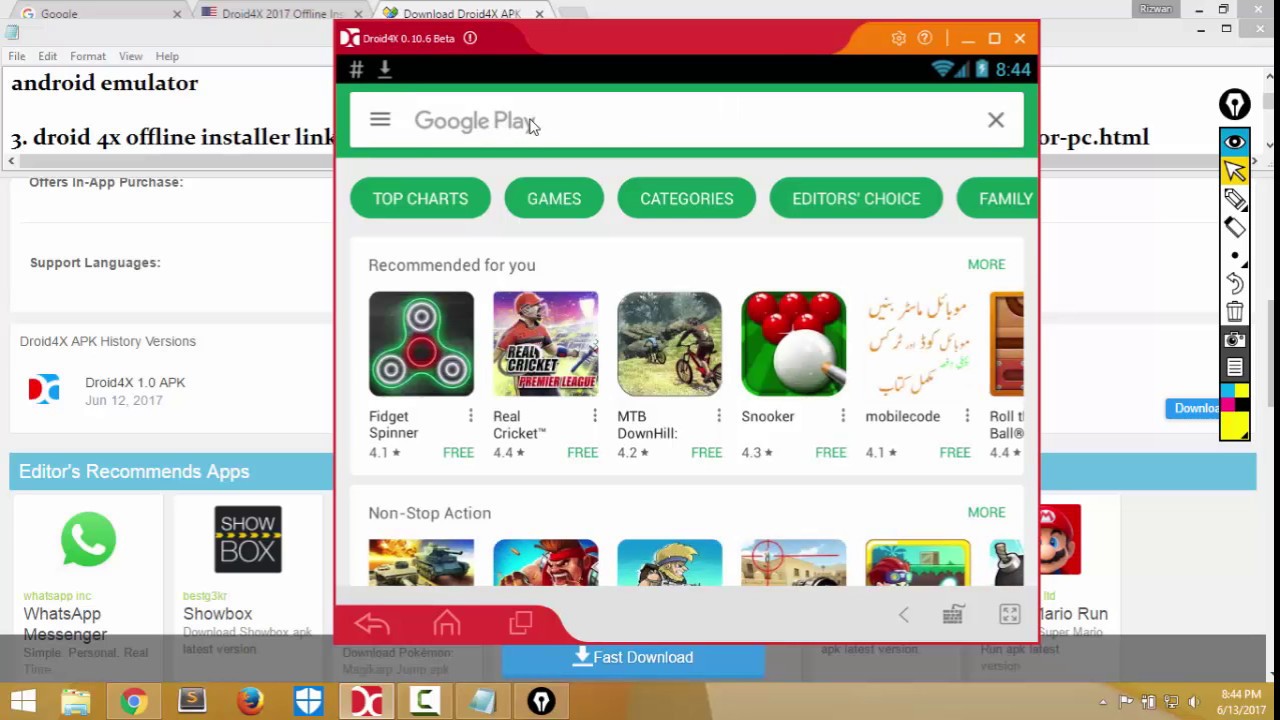This detailed horizontal image captures a screenshot from a desktop or laptop computer. At the top of the screen, there's a slender, elongated, gray rectangle displaying three browser tabs: a Google tab, a "Droid 4x2017 offline" tab, and a "Download Droid 4xAPK" tab. Situated vertically along the left-hand side are menu options labeled File, Edit, Format, View, and Help.

The main section of the screen features the title "Android Emulator," with a specific focus on the "Droid 4x offline installer link." Below this title, detailed information about the emulator is provided, including in-app purchase options, language support, and editor recommendations for apps such as WhatsApp, Messenger, and Showbox.

Embedded within this section is a secondary box displaying content from Google Play. This box includes tabs for Top Charts, Games, Categories, Editor's Choice, and Family. It also shows a grid of different game icons, each accompanied by their name, rating, and price (if applicable).

Beneath this, there is another white box offering details about various downloads and options, with a specific mention of "Mario Run" and a "Fast Download" option.

Finally, the bottom of the screen showcases the taskbar, filled with icons for different applications including Windows, Chrome, and Firefox on the left. On the right side of the taskbar, it displays the time (8:44 PM) and date (June 13, 2017), along with additional system icons.